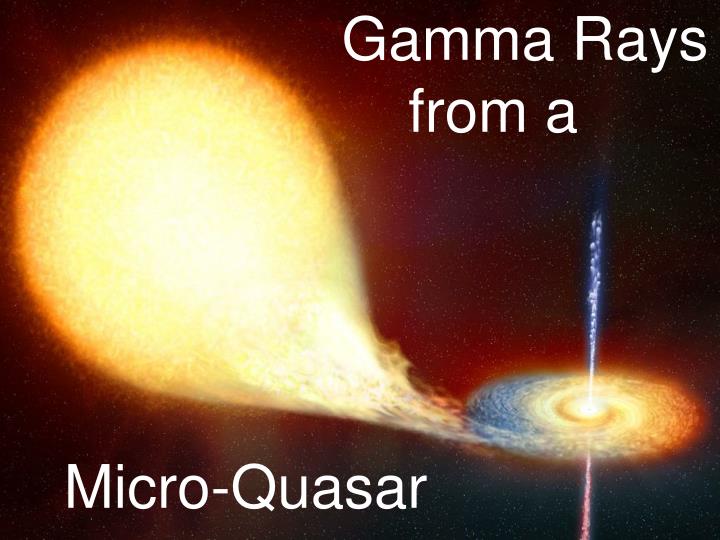The image appears to be a vividly captured view from space, likely a science poster demonstrating astronomical phenomena. Dominating the left side is an orange-red, somewhat circular fireball, resembling a comet or ballooning gas formation. Spanning from the top-right to the bottom-left, white text reads "gamma rays from A" and "microquasar," indicating the scientific context. The bottom right of the image displays a distinct spiral structure transitioning from orange-yellow to pronounced blue hues. This spiral includes a vertical stripe component visible at both the top and bottom. The entire composition suggests a spiral galaxy emitting or interacting with this fireball, embodied by swirling colors and a dramatic contrast between the energetic gamma rays and the quieter, spiral galaxy structure.